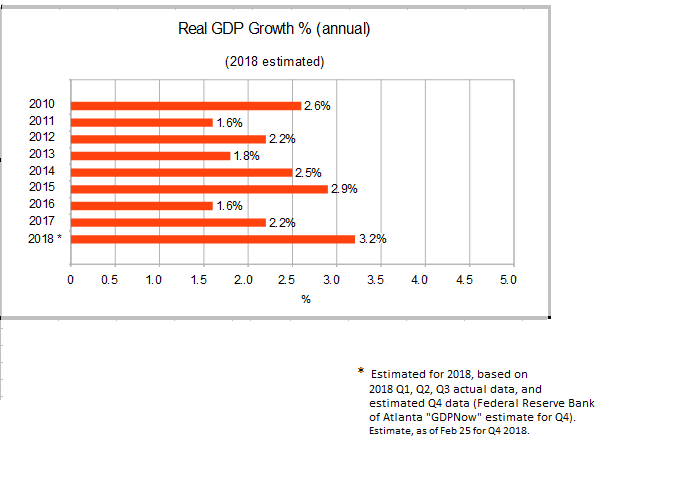This image presents a horizontal bar chart titled "Real GDP Growth Percent (Annual)", with a secondary title specifying "2018 Estimated". The chart tracks annual GDP growth from 2010 to 2018; each year is listed on the y-axis. The x-axis measures percentage growth from 0 to 5%, in 0.5% increments. Bar lengths represent the growth rates: 2.6% for 2010, 1.6% for 2011, 2.2% for 2012, 1.8% for 2013, 2.5% for 2014, 2.9% for 2015, 1.6% for 2016, 2.2% for 2017, and an estimated 3.2% for 2018, marked with an asterisk. The asterisk note explains the estimate is based on actual data from Q1 through Q3 of 2018 and estimated Q4 data from the Federal Reserve Bank of Atlanta’s GDPNow estimate as of February 25, 2018.